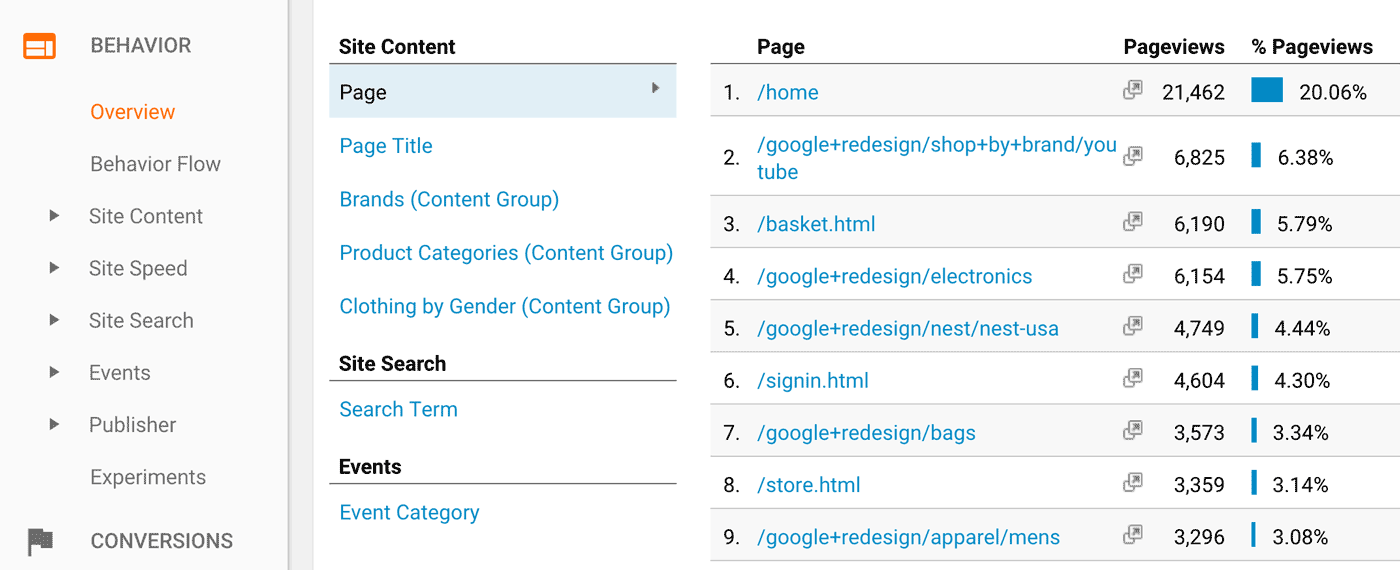The image displays an analytical dashboard focused on website behavior metrics. In the upper left corner, there's a heading labeled "Behavior" with a small orange box to its left. Adjacent to this on the right is the section titled "Site Content," which further breaks down into detailed categories. 

At the top, it lists "Page" and "Page Views," presenting the number of views for specific pages within the site. The detailed breakdown includes:

1. Home
2. Google Redesign
3. Basket
4. Google+ Redesign / Electronics
5. Google+ Redesign / Nest / Nest USA
6. Sign in HTML
7. Google+ Redesign / Bags
8. Store.html
9. Google+ Redesign / Apparel / Men's

Each page entry shows the number of page views and their respective percentages. The left section under "Site Content" also includes a mention of "Page Title," "Brands," "Product Categories," and "Clothing by Gender," providing a structured way to understand user interaction with the site’s content.